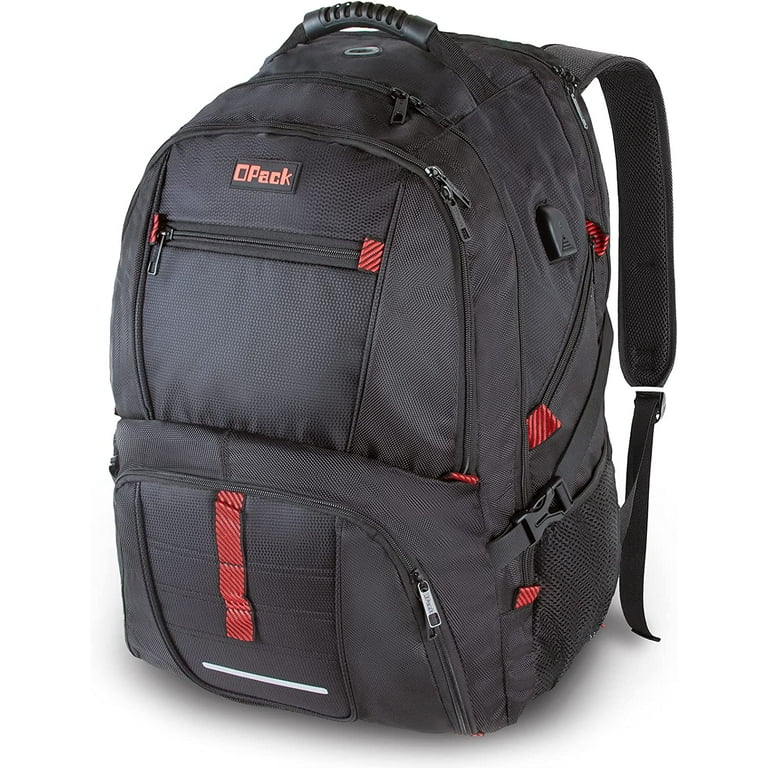This is a professional product photograph featuring a stocky black backpack with dark red accents, designed predominantly for hiking. The backpack appears robust and has considerable depth despite its moderate height. It is presented at a 45-degree angle, showcasing both the front and side, isolated against a pristine white background. The material of the backpack seems to be a durable vinyl nylon mix. The backpack features numerous compartments and zipper pouches, offering ample storage and organization options. Notably, every zipper is highlighted with a red tab. On the front, you can see a logo that reads "D-Pack," which may be the brand or model name. Additional details include a white horizontal line and several velcro straps, which may help secure additional items externally. There is also black netting on the side for holding items like water bottles, and the top of the backpack sports a black leather handle.